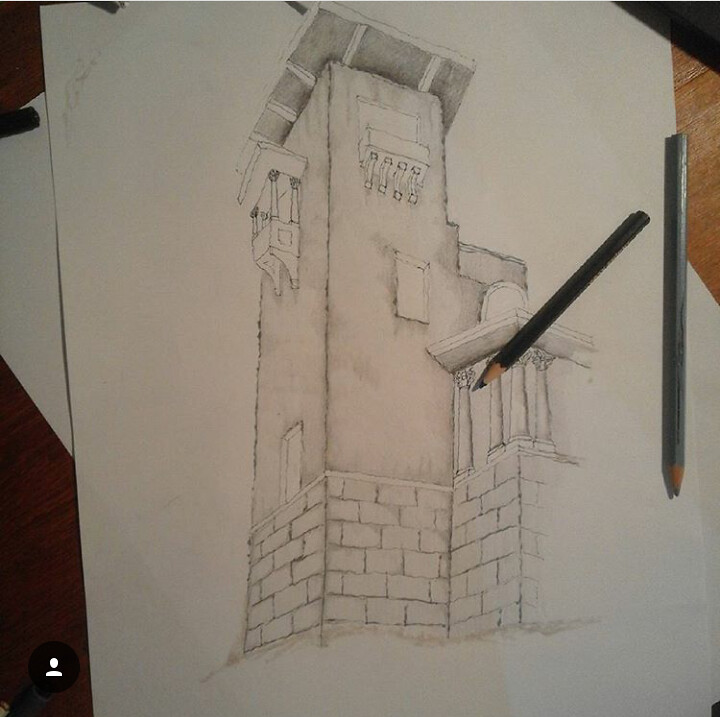This color photograph features a detailed line drawing of a tower, rendered in pencil. The drawing is displayed on several sheets of paper that rest on a brown wooden surface, which appears lighter on the left side and darker on the right. Distinctly visible at the bottom right of the image is a black logo, depicting the head and shoulders of a person in white.

The tower depicted in the line drawing reaches upward, with a perspective that looks towards the roof, adding a sense of height and grandeur. Detailing includes several lines traversing the roof, possibly representing architectural features such as trusses or support beams. Intriguingly, midsection embellishments suggestive of colors or levees add to the complexity of the structure.

The tower design features squarish windows on both the front and side elevations. One side window includes what appears to be a balcony on both the top and bottom, offering an extra layer of architectural intrigue. Near the base of the tower, rows of neatly aligned bricks give it a sturdy, robust appearance. A smaller tower is positioned in front of the main structure, similarly adorned with several rows of bricks.

Lastly, the composition is accented by two pencils casually placed on the drawing paper at the right-hand side, one black and the other gray, arranged diagonally and vertically, adding a touch of artist’s presence to the scene.